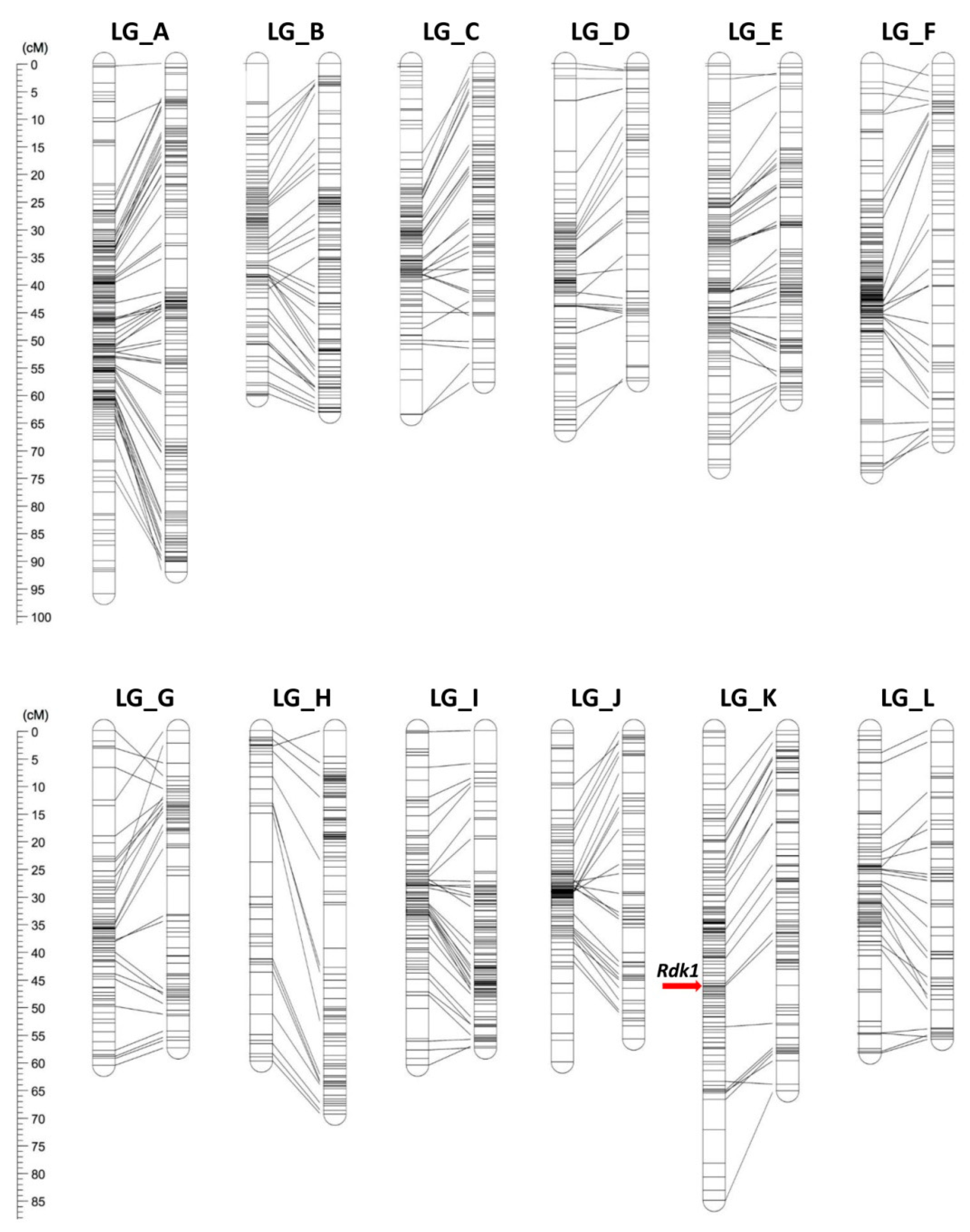The image showcases two intricate charts, one positioned above the other. Each chart features a vertical scale on the left-hand side, with the top chart's scale ranging from 0 to 100 and the bottom chart's scale going from 0 to 85. Both charts contain multiple sets of double columns labeled LG_A through LG_F on the top chart and LG_G through LG_L on the bottom chart. Each set of double columns is not uniform in size, with varying lengths and filled with different shades of color, indicating some form of measurement in centimeters. The columns are interconnected with multiple lines drawn in various directions, creating a complex web of patterns. Notably, in the LG_K section on the bottom chart, there is black writing to the left of the left column and a red arrow pointing towards it. Despite the detailed visual information provided, the charts lack any descriptive titles or instructions, leaving the precise nature of the measurements and their significance ambiguous.